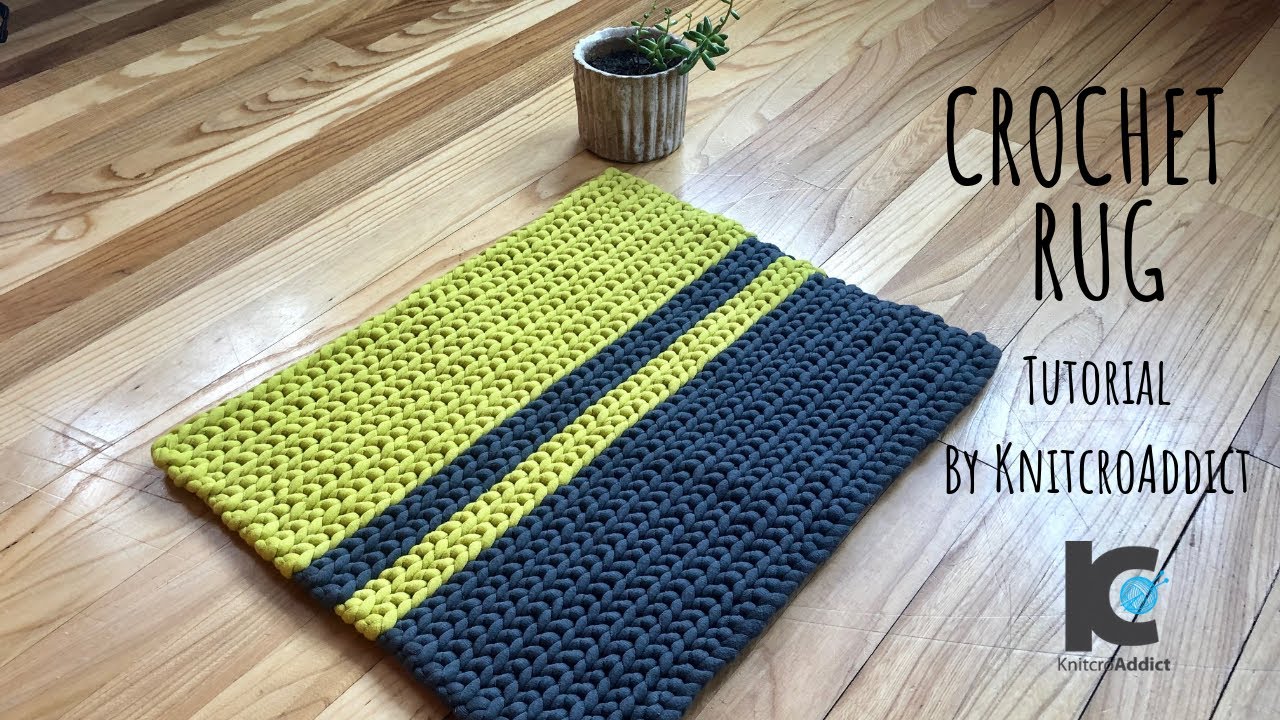The image features a well-crafted crocheted rug set on a slightly shiny hardwood floor with visible scratch marks. The rug itself is divided down the center, with the left side predominantly lime green featuring a double navy blue stripe near the center, and the right side mainly navy blue with a double lime green stripe, creating a mirror effect where the colors seem to switch sides. Above the rug sits a small, unidentified plant in a vertically-striped pot, which appears to be a succulent. To the right, text in a handmade-looking font reads "Crochet Rug," followed by "Tutorial by Knit Crow Addict," alongside a logo featuring an intertwined 'K' and 'C' with a blue sphere. Underneath, it repeats "Knit Crow Addict," reinforcing the brand identity. The overall composition suggests this is likely an advertisement or educational pamphlet for a crochet tutorial by Knit Crow Addict.